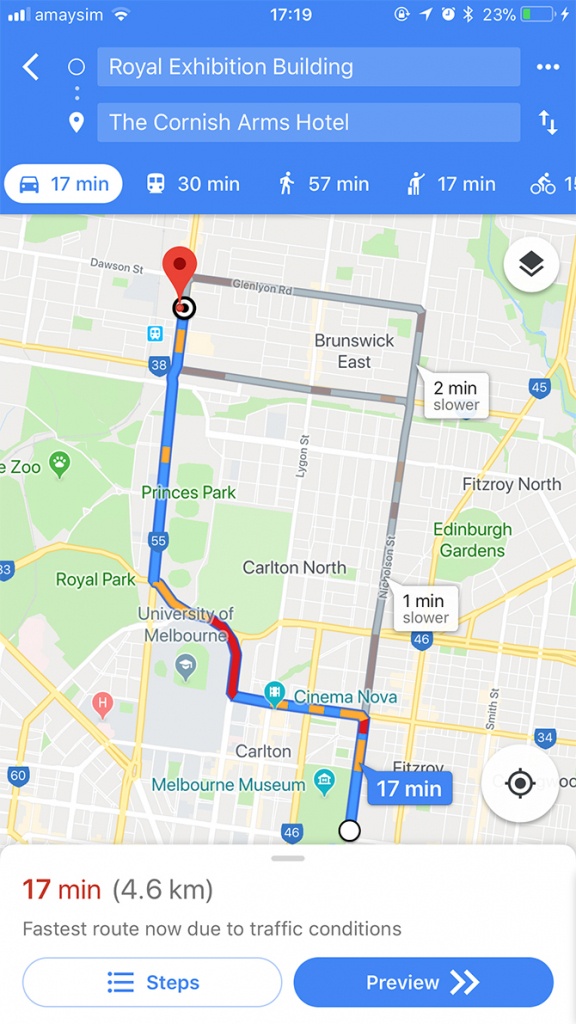### Descriptive Caption:
A mobile screenshot from an Android phone displaying Google Maps navigation. The device is connected to the Amaysim cellular network with three out of four signal bars and has two out of three Wi-Fi bars. The status bar shows the current time as 17:19, with rotation lock, location services, a set timer, and Bluetooth all active. The battery level is at 23% but is currently charging.

The screenshot details a navigation route from the Royal Exhibition Building to the Cornish Arms Hotel. The estimated travel times are 17 minutes by car, 30 minutes by public transport, 57 minutes by walking, and 17 minutes by rideshare services like Uber or Lyft, with an alternative longer time for biking. The user has chosen to drive, with the distance noted as 4.6 kilometers taking approximately 7 minutes.

Various points of interest are marked on the map, including the Melbourne Zoo, Prince's Park, Royal Park, Brunswick East, Carlton North, University of Melbourne, Melbourne Museum, Carlton, Cinema Nova, Fitzroy, and Edinburgh Gardens. A notification at the bottom of the screen indicates that the current route is the fastest available due to traffic conditions, with options to view steps or a route preview.

Overall, this image captures the detailed navigation interface of Google Maps as the user plans their journey.